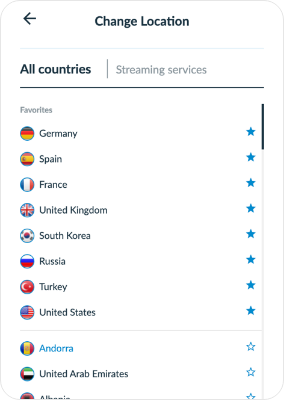The image features a simple user interface design against a white background. At the top-center, prominent black bold text reads "Change Location," accompanied by a left-pointing black arrow beside it. Directly below, the text "All Countries" is displayed, with "Streaming Services" in gray aligned to the far right. A black horizontal line separates this header section from the rest of the content.

Below the line, the section labeled "Favorites" introduces a column of country flags on the left. The respective country names are positioned to the right of each flag. To the far right of each country's name is a blue star. The countries listed in descending order are:

- Germany
- Spain
- France
- United Kingdom
- South Korea
- Russia
- Turkey
- United States

Following these entries, the list continues with the stars retaining blue edges but featuring white centers. In this section, "Andorra" is distinctly written in blue text, followed by "United Arab Emirates." The remainder of the image is largely unoccupied, consisting of empty white space.